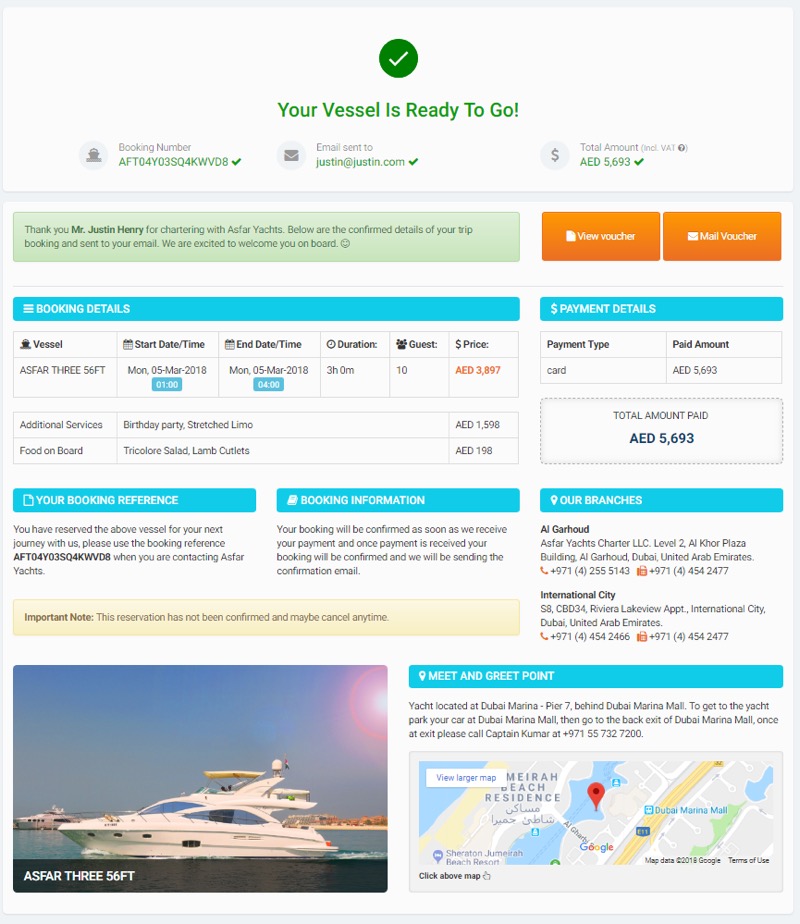This image is a screenshot from a cruise booking website. The background is predominantly white, with a green circle featuring a white checkmark at the top center. Directly beneath the circle, in green text, it reads, "Your vessel is ready to go!" followed by an exclamation mark. The payment summary below indicates that the person has paid 5,693 AED. 

On the left side, there is a sky blue banner with the text "Booking Details" in white. The detailed information provided includes the name of the vessel, the start date, and the end date of the cruise. At the bottom left corner, there's an image of a sleek, small ship labeled "ASFAR 356FT." 

On the lower right-hand corner, there is a map displaying the meet and greet point, marked with an inverted red teardrop.